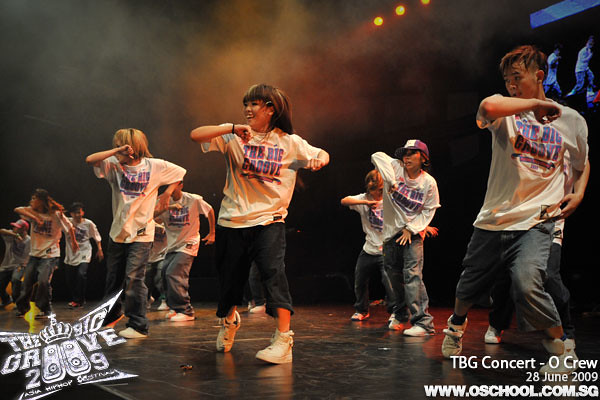The image depicts a dynamic indoor scene featuring several young individuals dancing on a stage. The performers are dressed in matching white t-shirts with a blue logo that reads "The Big Groove." They appear to be engaged in a synchronized dance routine, all striking similar poses with their right arms bent near their faces and their left arms down by their sides. The stage is centrally positioned within the frame, and the background is dark, illuminated by overhead lighting. In the bottom left corner, there is a white logo with a crown that says "The Groove 2009." Additionally, white text in the bottom right corner reads "TBG Concert, O School, June 28, 2009, www.oschool.com.sg." A screen or reflection is visible in the upper right corner. The photograph, shot in landscape orientation, captures the essence of a vibrant concert performance, with the date and event details prominently displayed. The setting appears to be indoors, focusing on the dancers' energetic movements and the overall lively atmosphere.